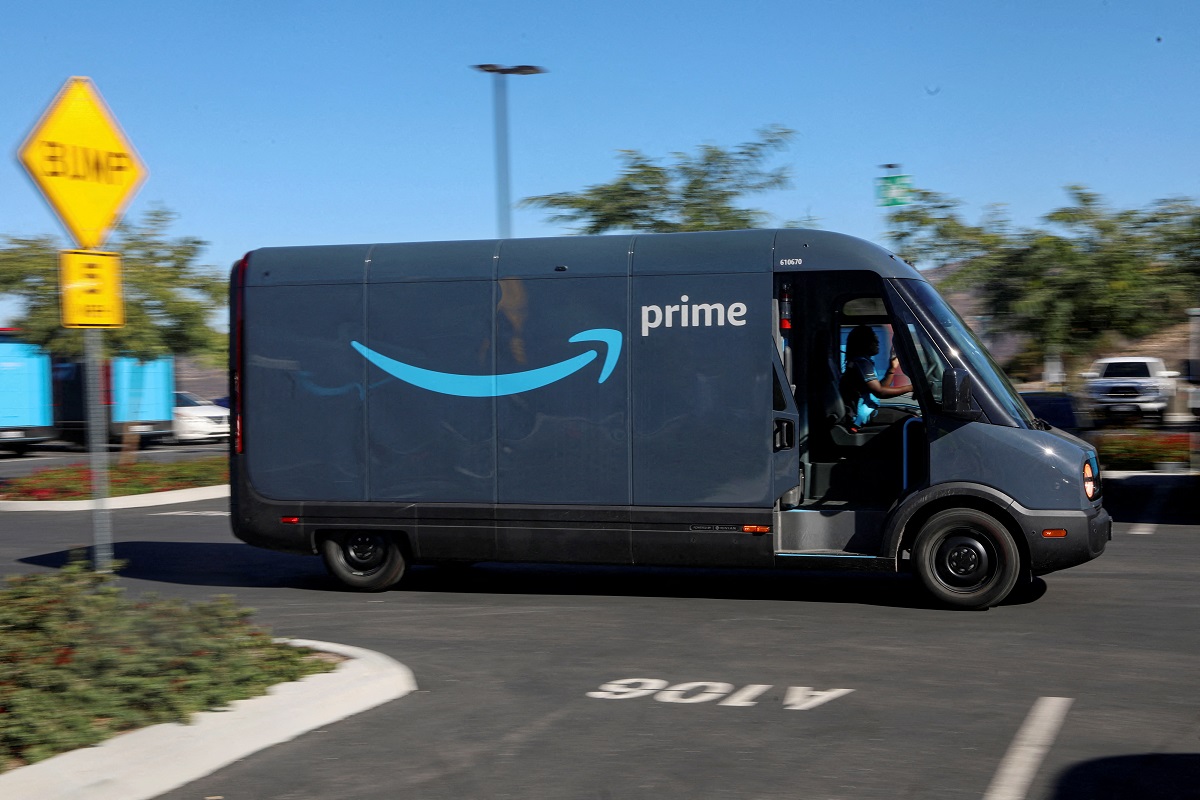The photograph captures an Amazon delivery truck prominently positioned in the center of the frame, with the front of the vehicle facing towards the right. The truck is approximately two inches from the right and left edges of the image. The vehicle features black wheels and rims, with its body enveloped in a dark blue color that extends across the sides, top, and front hood. The back of the truck sports a black section with a black border underneath. 

A large window at the front reveals a person sitting inside, and there is no door, allowing a clear view into the gray area where one steps into the truck. On the side of the truck, prominently displayed is a big blue Prime check mark, with the word "Prime" in white at the check's point.

The background features a clear blue sky. To the left of the truck, a tree is visible alongside two other Amazon Prime trucks, light blue in color, and the back of a white car. Adjacent to these vehicles, there is a yellow road sign indicating a bump ahead, mounted on a silver pole, featuring red, white, and black lettering.

In the bottom left corner of the photo, greenery and a curb painted gray are present. The Amazon truck sits parked on a gray paved road, with a parking spot labeled "A106" visible below it. A white line marking lane divisions runs off to the right of this parking spot, and a faint shadow can be seen in the right corner.

Above the truck, a portion of a light pole and a small section of a tree come into view. Further to the right, another tree stands nearby, and a white truck is noticeable off in the distance, beyond which are rows of bushes lining a white-painted curb.